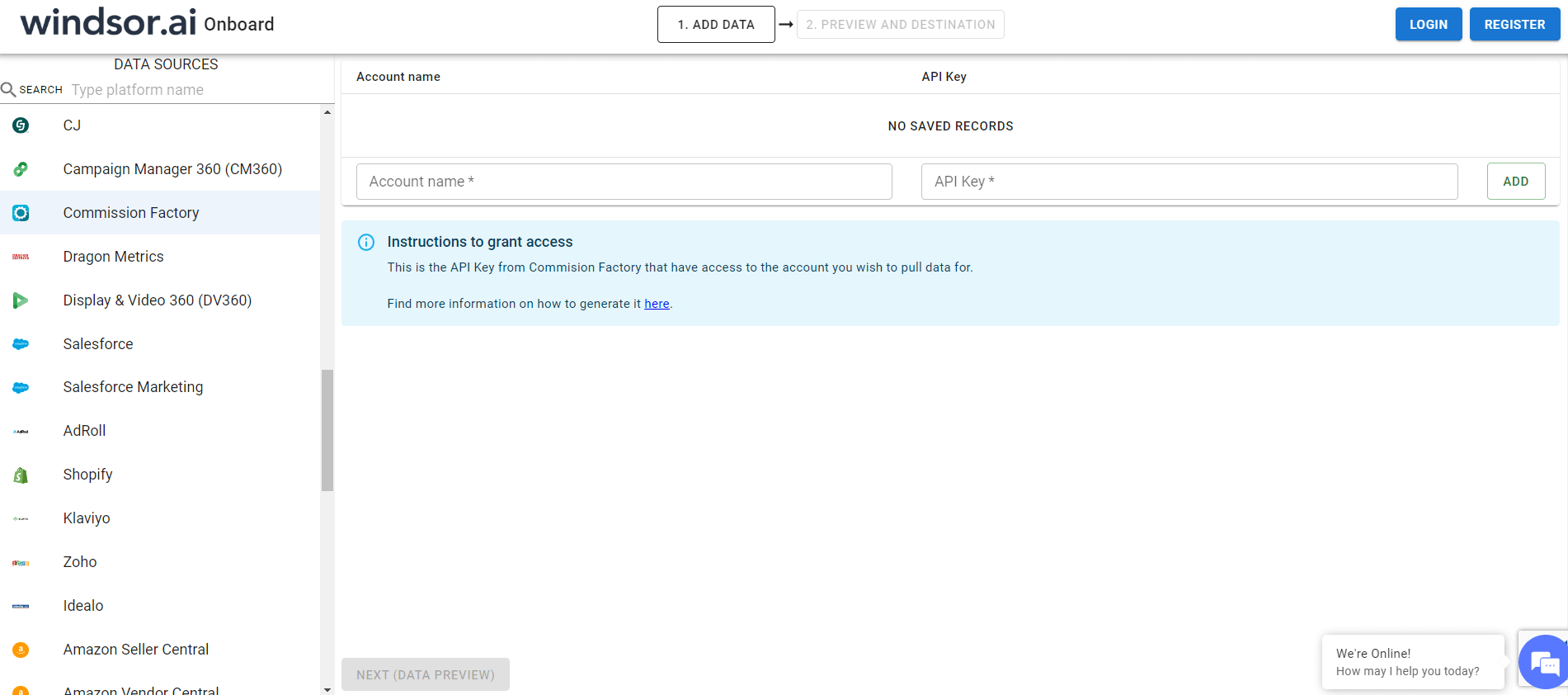**Detailed Caption:**

This screenshot illustrates the interface of the Windsor.ai application or website, specializing in AI-driven services. The top left corner prominently displays the Windsor.ai logo. The navigation bar at the top row features two primary buttons: "Add Data", which is highlighted as the first step, and "Preview and Destination", which is grayed out, indicating it is not yet accessible. To the far right of the top row, there are two separate buttons labeled "Login" and "Register".

On the left-hand side, a vertical column labeled “Data Sources” is visible. Within this column, a search box prompts users to "Type platform name." Below the search box, a list of data services is presented, including CJ, Campaign Manager 360, Commission Factory, Dragon Metrics, Display & Video 360, Salesforce, Salesforce Marketing, Adpole, Shopify, Klaviyo, Zoho, Idealo, Amazon Seller Central, and Amazon Vendor Central. The presence of a scroll bar suggests there are additional options not visible in this screenshot.

To the right of the “Data Sources” column, there are input fields for "Account Name" and "API Key," with a notification stating "No saved records." Users are required to input their account name and API key to access further functionalities. Once these fields are populated, the user can click the "Add" button located to the far right of the input boxes. 

Currently, since no data has been input, a blue highlighted box titled "Instructions to Get Access" is displayed. This box includes specifics on obtaining the API key from Commission Factory, with a hyperlinked "here" for more detailed instructions on generating this key.

At the bottom of the interface, a grayed-out button labeled "Next Data Preview" indicates that the next step is not yet available. In the bottom right corner, a small chat bubble pops up with the message, "We're online. How may we help you today," offering immediate assistance.